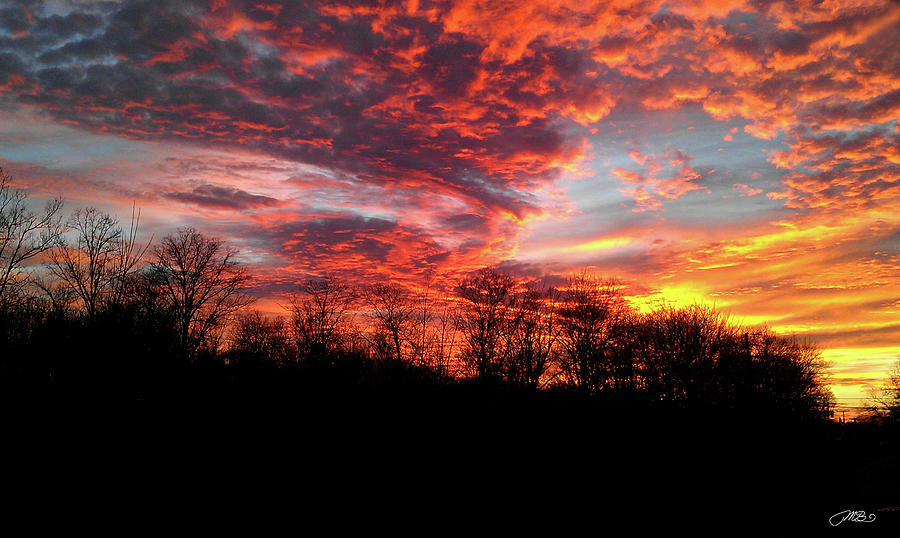This photograph captures a stunning sunset with a dramatic sky and a distinctive tree line. The bottom half of the image is a solid black silhouette of leafless trees, indicative of late fall or early winter. Above, the sky transitions from light, bright orange and pink clouds near the horizon, where the sunset occurs, to darker pink and purple hues as you move leftward across the image. The sunset appears near the bottom right of the photo, casting a warm glow and creating a small, bright yellow area surrounded by rich orange and pink accents. The sky displays a blend of colors, with cyan and blue streaks intermingling with the vibrant clouds. The entire upper portion of the sky is a mix of dark purple, blue, and light orange clouds, composing a breathtaking mosaic. At the bottom right, a small white signature, possibly the photographer's, subtly marks the image. The overall contrast between the dark, bare trees and the colorful, illuminated sky adds to the photograph's striking beauty.